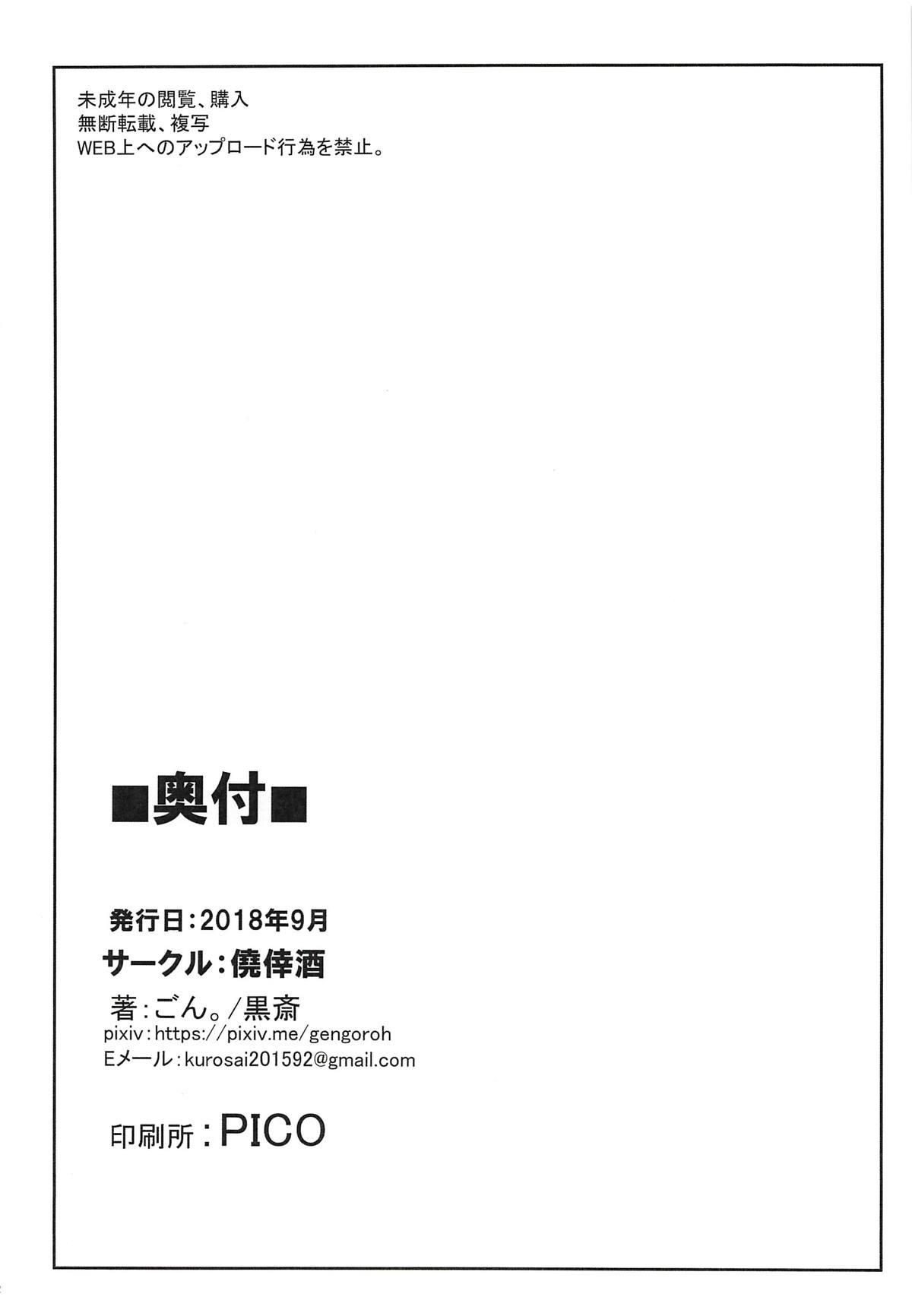The image features a stark white background with all the text enclosed within a thin black rectangular border, resembling a photocopy or a printout of some sort. In the upper left and bottom left corners, there are lines of Japanese text. Prominently in the bottom left corner, the text "PICO" is displayed along with the year "2018", and further down, there are URLs and contact information. One URL reads "pixiv.me.gangaro" and the email address is "kurosai201592@gmail.com." Additionally, there is a shadow visible in the top right corner suggesting the image was scanned from a sheet of paper. The overall layout hints at a letterhead or contact form.